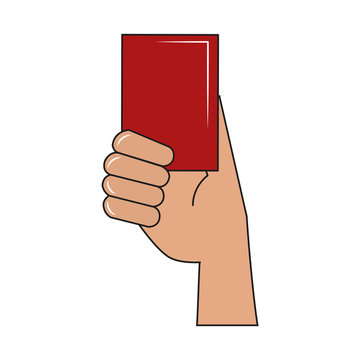This simplified, cartoon-style image features a right hand drawn in a clipart fashion, set against a pure white background. The hand, shown from the side with only four fingers visible and the thumb obscured behind a red rectangle, appears to be holding a red object that could be a wallet or card. The red object is accentuated with a white line forming a 90-degree corner at the top right, possibly to simulate light or shadow. The outlines of both the hand and the red object are defined with black lines, contributing to the clipart aesthetic. The image ends at the wrist, positioned at the bottom right-hand corner.